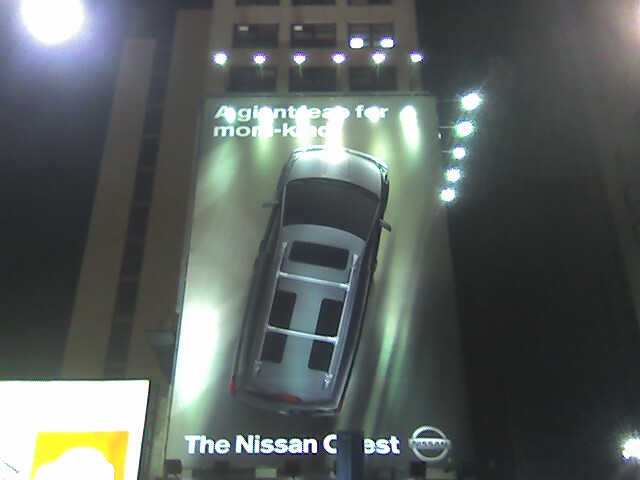In this somewhat blurry nighttime image, a large, illuminated billboard is prominently displayed against the side of a tall, tan-beige skyscraper, which could be either an apartment building or a downtown office structure. The billboard features a top-down view of a car with some sun glare effects, accompanied by the partially obscured text—possibly reading “Asian for mom” or something similar—due to light reflections. The bottom right corner of the billboard clearly shows the Nissan logo along with the model designation, likely “Nissan C-est.”

In the upper left corner of the image, a round moon is visible, adding to the night ambiance. The bottom left corner shows a washed-out sign, predominantly white with some yellow elements, whose details are lost in the glare. Additional street lights and a hazy light effect can be seen in the bottom right corner, and a faint, colorful light haze appears in the upper right corner of the image.